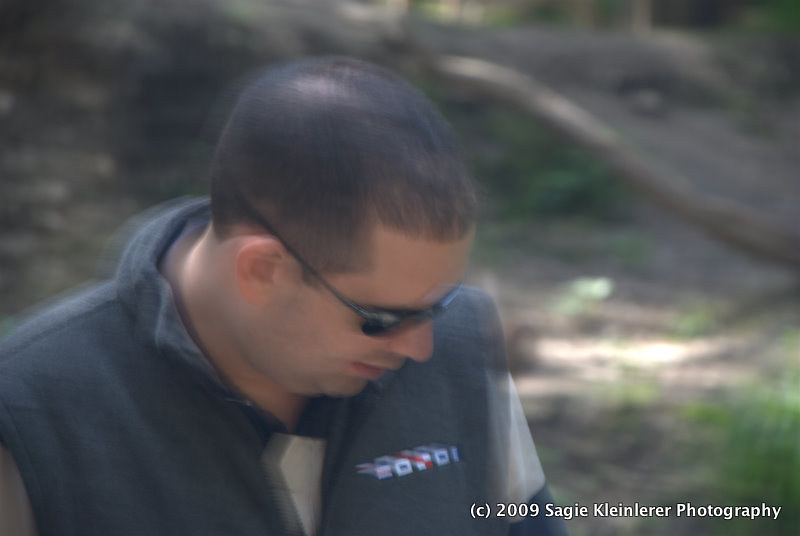A blurry image captures a Caucasian man wearing sunglasses and looking down, possibly at his feet, as he traverses through a forest. The ground is sandy with sporadic patches of grass and weeds. He is dressed in a blue zip-up jacket featuring markings on the left chest, which might be decorative rather than medals. Underneath, he wears a white and blue striped shirt. The man sports a very short haircut. The forest behind him appears dense, with minimal sunlight filtering through, and to the right, there's a fallen log near what looks like a ravine.